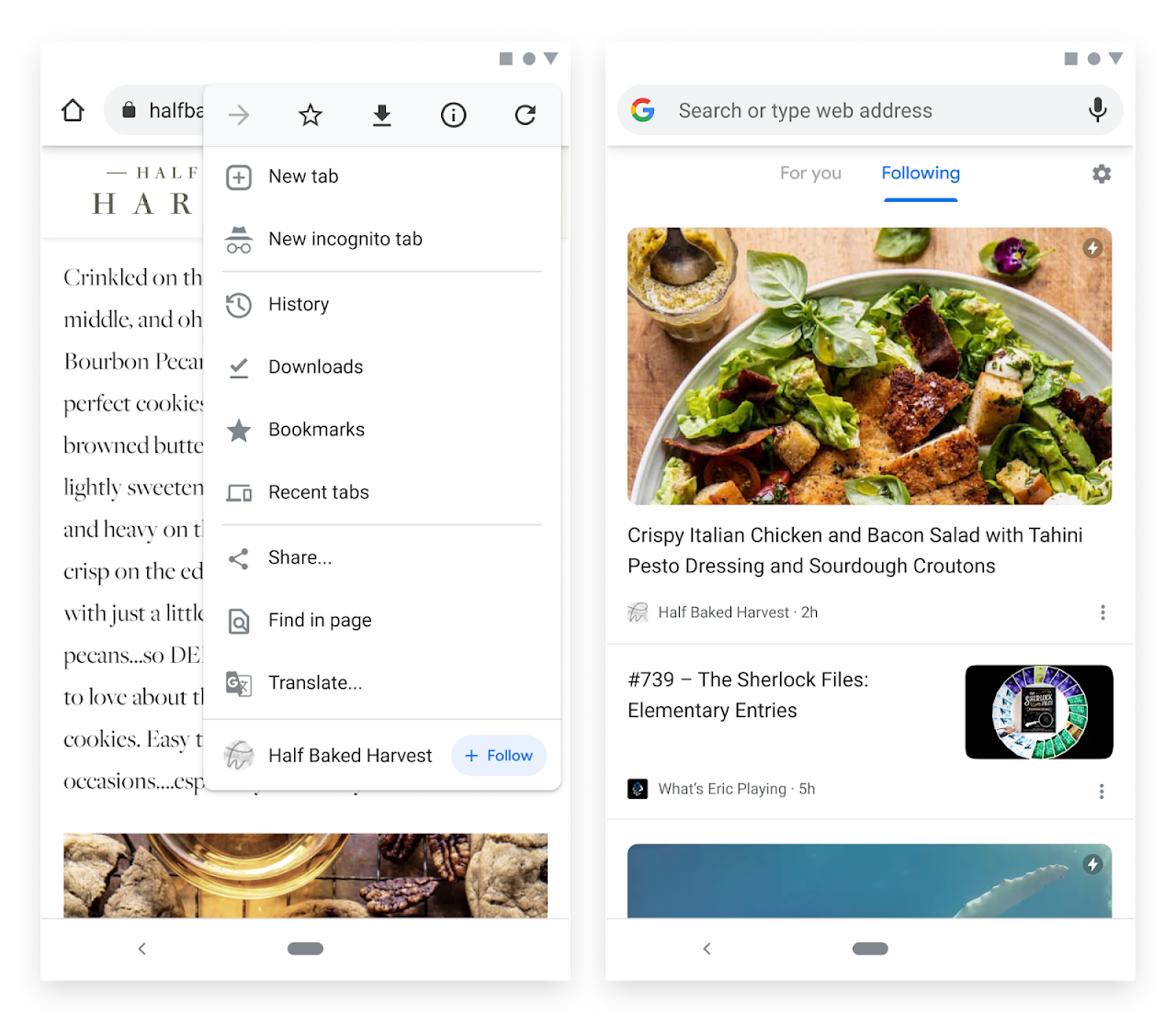**Detailed Caption:**

The image showcases two side-by-side screenshots captured from a cell phone, each presenting a distinct section of a web page with notable similarities and differences.

On the left screenshot, the top portion features a consistent white background with three gray shapes: a square, a circle, and a down arrow. A pop-up window partially obscures the URL bar, showing only a gray padlock, a gray home button, and the text "half BA" just outside the pop-up. This pop-up is a familiar Google Chrome browser menu, displaying options like "New Incognito Tab," "History," "Downloads," "Bookmarks," and "Recent Tabs," among others. Above the menu are the typical browser icons: a right arrow for navigation, a star for bookmarks, a download button, an information button, and a reload button. The content beneath the pop-up suggests a recipe or meal description interface, highlighted by fragmented text in gray and black on a white background. The website, "Half-Baked Harvest," is somewhat visible with a Follow button integrated into the Google Chrome menu button. The partially visible imagery behind the pop-up hints at a barbecue grid with charcoal and food items being grilled.

The right screenshot similarly starts with a white background, a multicolored Google "G" on the left of the search bar, and a gray microphone icon on the right. Top left features gray text reading "For You," with the blue word "Following" underlined on the right. A gray gear icon sits in the upper right corner. Below, an appetizing image of a chicken salad in a white bowl catches the eye. Beside the salad is a drink in the upper left corner, placed on a wooden table. The black text underneath describes the dish as "Crispy Italian Chicken and Bacon Salad with Tahini Pesto Dressing and Sourdough Croutons," with "Half-Baked Harvest" stated in gray at the bottom left. Three vertical dots sit next to this description. Further down, another section titled "The Sherlock Files, Elementary Entries" is visible, next to the number 739. The right shows a multicolored-edged dinner plate with the text "What's Eric Playing? Five Hours" underneath in gray. The image on the bottom depicts a sky scene with white clouds and a white lightning bolt within a blue circle in the upper right.

This comprehensive portrayal combines both visual and textual elements to give a clear sense of the web pages depicted in the cell phone screenshots.